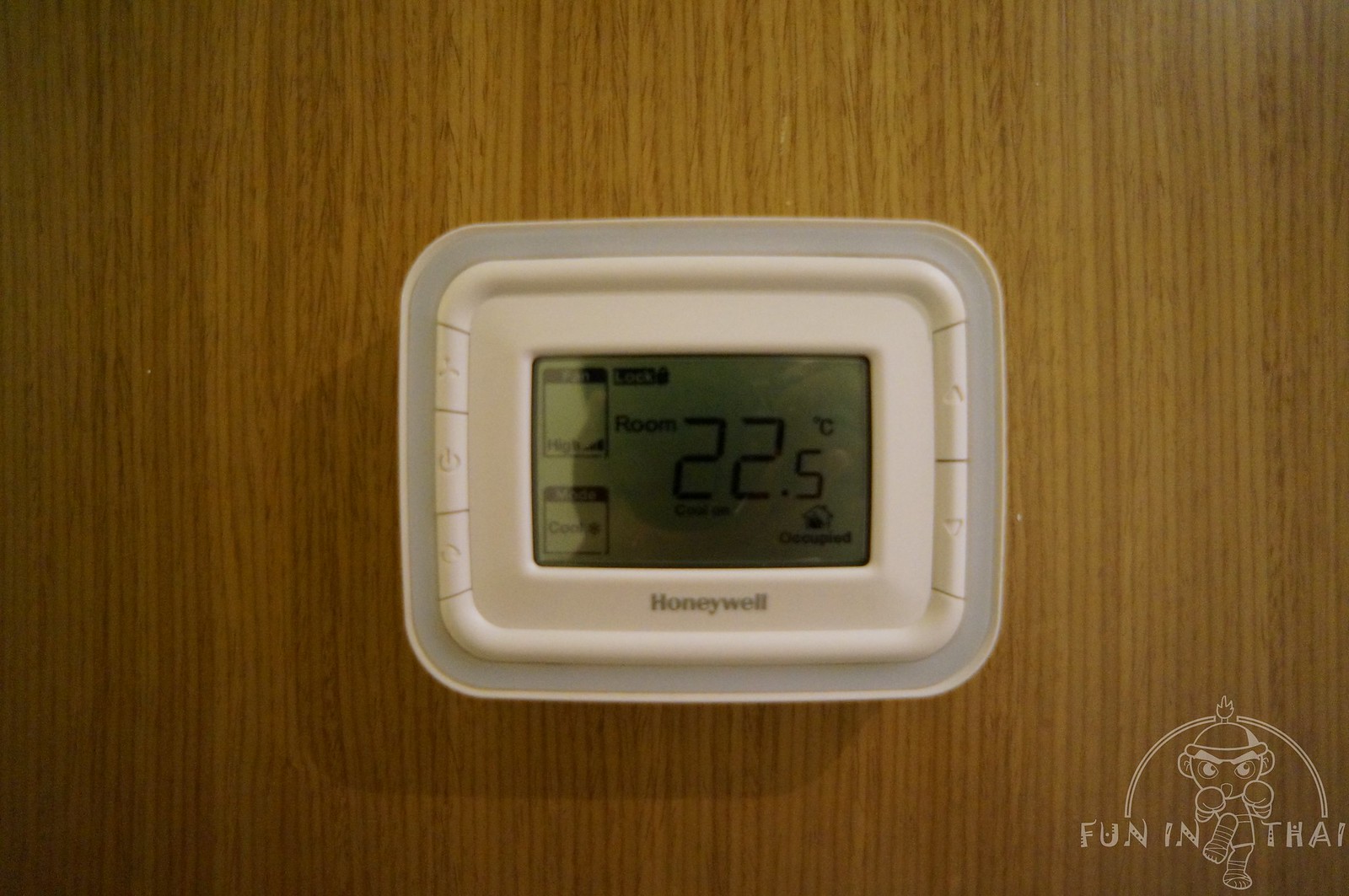The photograph features a Honeywell electric thermostat mounted on a wall with a light brown wood grain texture. The wall covering resembles bamboo, characterized by its vertical lines with occasional deviations, confirming it is indeed a textured wood grain rather than compressed cardboard. 

The white plastic thermostat, nearly square in shape but technically a rectangle, prominently displays the Honeywell logo in silver near its bottom. At the center of the device is a grey LCD screen showing the current room temperature as 22.5 degrees Celsius and indicating the status as "Occupied." Integrated buttons are subtly positioned along the device's edges, designed to blend seamlessly with the rest of the thermostat's casing.

In the bottom right corner of the image, there is a playful element – the word "Fun" in Thai, accompanied by a cartoon-like, chibi-style rendering of a Thai boxer. The boxer is depicted facing the viewer with hands up and one knee raised, capturing the dynamic essence of Thai boxing. The illustration is rendered in white, contrasting sharply against the background to draw attention despite its small size.